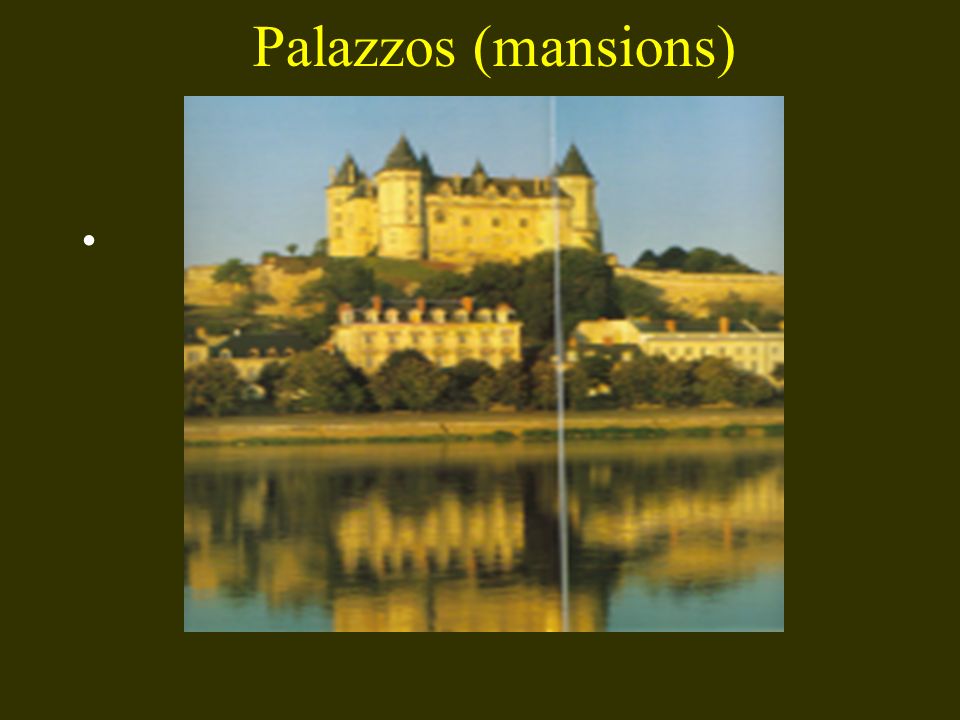The image depicts an old, somewhat blurry photograph of a large, white castle perched on a hill. The castle is characterized by four prominent steeples with round, pointy roofs, one at each corner, constructed from stone or cement. Below the castle, the hill descends to reveal three large structures resembling mansions, distinguished by their white, golden-yellow hue, black roofs, and orange chimneys. In the foreground of the image, there is a body of water, which could either be a pond, lake, or stream, accompanied by rows of green and yellow trees that line the housing complex. Additionally, the image appears to be a part of an educational slide, with olive green as the background color. At the top, in yellow text, it reads "Palazos" with the translation "(mansions)" in parentheses, suggesting the content might be utilized for language instruction.